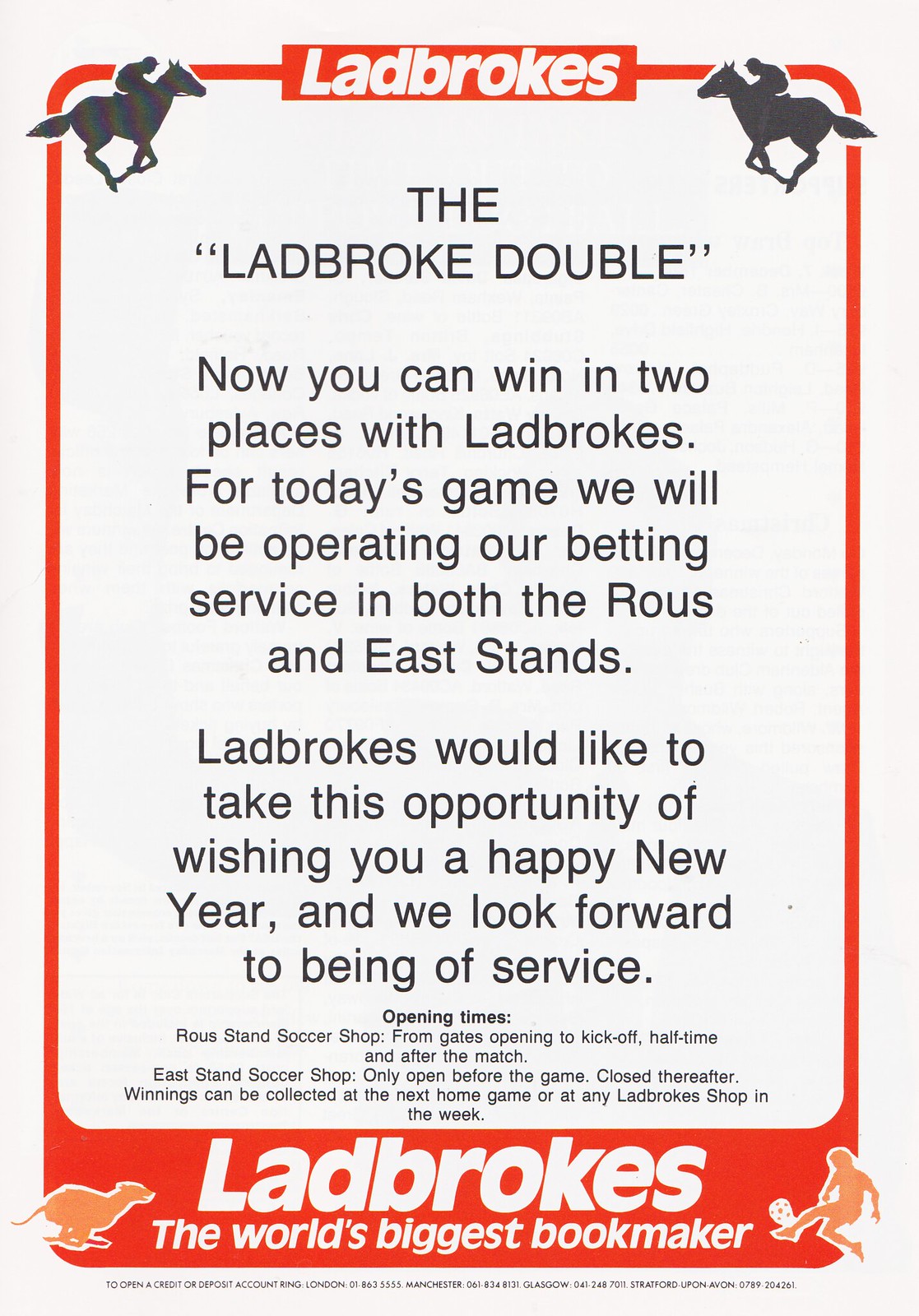The image is an advertisement for Ladbrokes, predominantly white with a distinctive red border that frames the content. At the top center, "Ladbrokes" is prominently displayed in bold white text set against a red background. Flanking the text on both the left and right are black silhouettes of horses with jockeys, converging towards the center.

In the middle of the image, the text reads: "The Ladbroke Double. Now you can win in two places with Ladbrokes. For today's game, we will be operating our betting services in both the Rose and East Stands. Ladbrokes would like to take the opportunity of wishing you a Happy New Year, and we look forward to being of service." Below this, additional information in smaller black text details the opening times: "Rose Stand Soccer Shop, from gates opening to kickoff, halftime, and after the match. East Stand Soccer Shop, only open before the game, closed thereafter. Winnings can be collected at the next home game or at any Ladbrokes shop in the week."

At the bottom of the image, another red section features "Ladbrokes" in large white font, accompanied by the tagline "The World's Biggest Bookmaker." On either side, there are orange silhouettes—a greyhound racing dog on the left and a soccer player kicking a ball on the right. There is also very small black text beneath these elements, too minute to be legible.